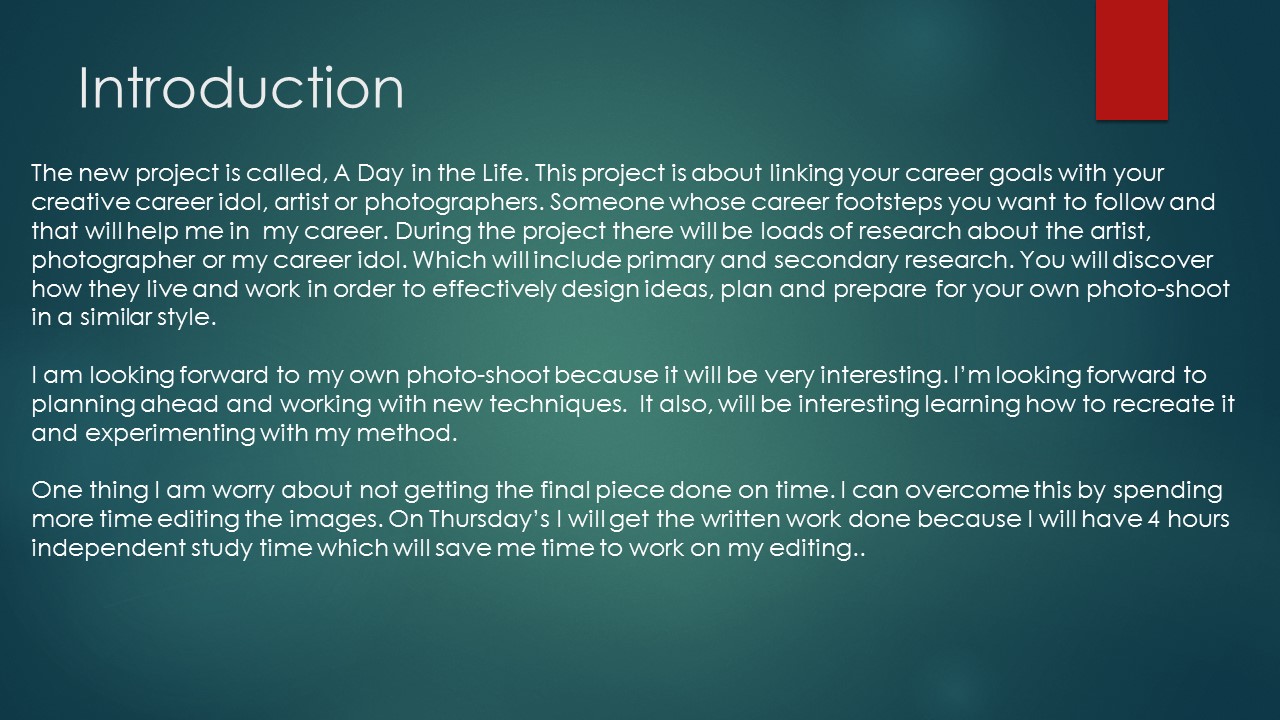The slide from the presentation features a dark teal background that lightens toward the center, with a small red rectangle in the top right corner. In bold white text on the upper left, it reads "Introduction." Below this heading, there are three detailed paragraphs explaining a new project called "A Day in the Life." This project aims to align your career goals with those of your creative mentor—whether an artist, photographer, or career idol—whose path you aspire to follow in order to aid your own career progression. 

The project involves extensive research into the chosen mentor's life and work, incorporating both primary and secondary sources. This research will help you understand how they lived and worked, enabling you to design a comprehensive plan for the year or prepare for a photoshoot that emulates their style. The text expresses excitement about the prospect of conducting a personal photoshoot, planning ahead, and utilizing new technologies. It also highlights the anticipation of learning to recreate and experiment with different methods. A concern is noted about not completing the final piece on time; however, a solution is proposed—dedicating Thursdays to writing tasks during a four-hour independent study period, freeing up time for editing the images.